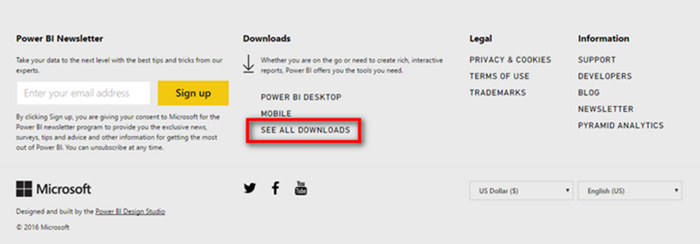Here's a more detailed and cleaned-up descriptive caption for the image:

---

This image is a cropped screenshot of a website or application footer, featuring a light gray background and divided into two main sections. 

### Top Section:
**Column 1:**

- **Heading (Bold, Black Sans-Serif, Title Case):** Power BI Newsletter
- **Description Text (Small Font):** "Take your data to the next level with the best tips and tricks from our experts."
- **Email Subscription Field:** A field for entering your email address accompanied by a yellow button labeled "Sign Up" in black letters.
- **Consent Text (Small Font):** "By clicking Sign Up, you are giving your consent to Microsoft to the Power BI Newsletter program to provide you with exclusive news, surveys, tips, and advice. You can unsubscribe at any time."

**Column 2:**

- **Heading (Bold, Black Sans-Serif):** Downloads
- **Icon:** Download icon featuring an arrow pointing down at a line.
- **Description Text (Paragraph):** "Whether you are on the go or need to create rich interactive reports, Power BI offers you the tools you need."
- **Links (All Capitals, Black Letters):**
  - Power BI Desktop
  - Mobile
  - See All Downloads

**Column 3:**

- **Heading (Bold, Black Sans-Serif):** Legal
- **Links (All Capitals, Black Letters):**
  - Privacy and Cookies
  - Terms of Use
  - Trademarks

**Column 4:**

- **Heading (Bold, Black Sans-Serif):** Information
- **Links (All Capitals, Black Letters):**
  - Support
  - Developers
  - Blog
  - Newsletter
  - Pyramid Analytics

**Note:** The screenshot displays an edited element, a red rectangle with a shadow hovering over it. This appears to have been added manually rather than being part of the actual website or application.

### Bottom Section:
**Column 1:**

- **Logo and Description:** Microsoft logo with the text "Designed and built by the Power BI Design Studio © 2016 Microsoft."

**Column 2:**

- **Social Media Icons:** Twitter, Facebook, and YouTube.

**Column 3:**

- **Drop-down Menus:** Two drop-down menus displaying "US Dollar" and "English (US)" respectively.

---

This caption provides a comprehensive description of the footer, ensuring that every element is detailed and organized for clarity.